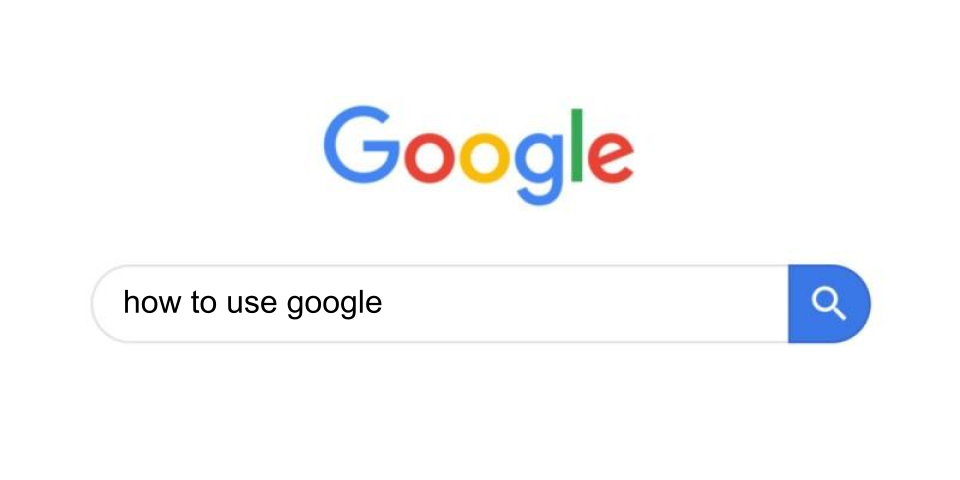The image displays a segment of a webpage, showing a traditional Google search interface. The background is entirely white, allowing the central elements to stand out prominently without distraction. At the top of the image, the word "Google" is presented in large, multicolored letters, adhering to Google's recognizable color scheme: the first capital "G" in blue, the first "o" in red, the second "o" in yellow, the lowercase "g" in blue, the "l" in green, and the "e" in red. The font used is Google's distinctive sans-serif typeface.

Beneath this vibrant logo, a sleek, elongated oval-shaped search bar is positioned horizontally. The search bar is outlined by a thin gray line, adding subtle definition against the white background. On the extreme right end of the search bar, a blue shaded area matches the color of the two "G's" in "Google" and contains a white magnifying glass icon, indicating the search function.

Inside the search bar, the text "how to use google" is written in a black, all-lowercase, sans-serif font reminiscent of Arial. The rest of the space around these elements remains a clean, uncluttered white, directing full attention to the Google logo and the search bar, which dominates the scene.